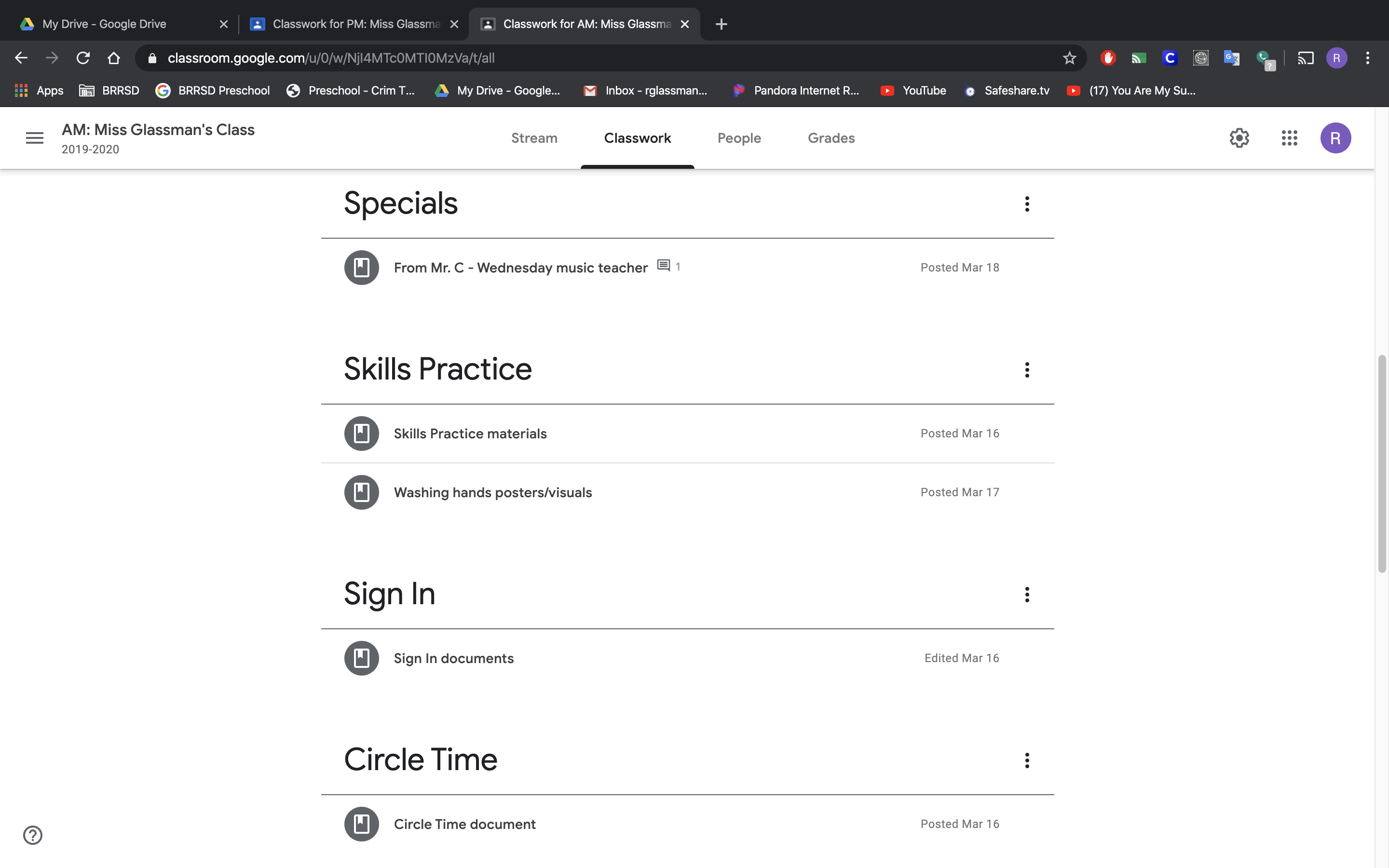A detailed screenshot of a desktop browser showcases a page with a white background body, accentuated by a white header above it, and topped by a dark gray browser header. The browser features a dark gray hamburger menu on the left side of the white header. To the right of the hamburger menu and slightly elevated, bolded black text reads "AM: Miss Glassman's class." Directly underneath, light gray text denotes the academic year, "2019 to 2020."

Further right, separated by a significant negative space, light gray text labels sections of the page: "stream," followed by black text "classwork" underlined in black, then "people," and "grades," both in light gray.

Toward the far right, another large empty space leads to icons: a light gray cogwheel, a light gray three-by-three grid of dots, and a purple circle with a white capital "R." A medium gray shadow appears beneath this section, emphasizing the transition to the body of the page.

In the top left of the main page area, large black text reads "specials." Below this, a medium gray thin line runs halfway across the page, centered. Beneath the line on the left, a dark gray circle encases a white icon depicting a piece of paper with a white bookmark at the top left. Adjacent to this is black text stating "From Mr. C - Wednesday music teacher." Continuing right, a dark gray comment icon containing three dark gray lines sits next to a light gray number "1," completing the visual elements of the page.